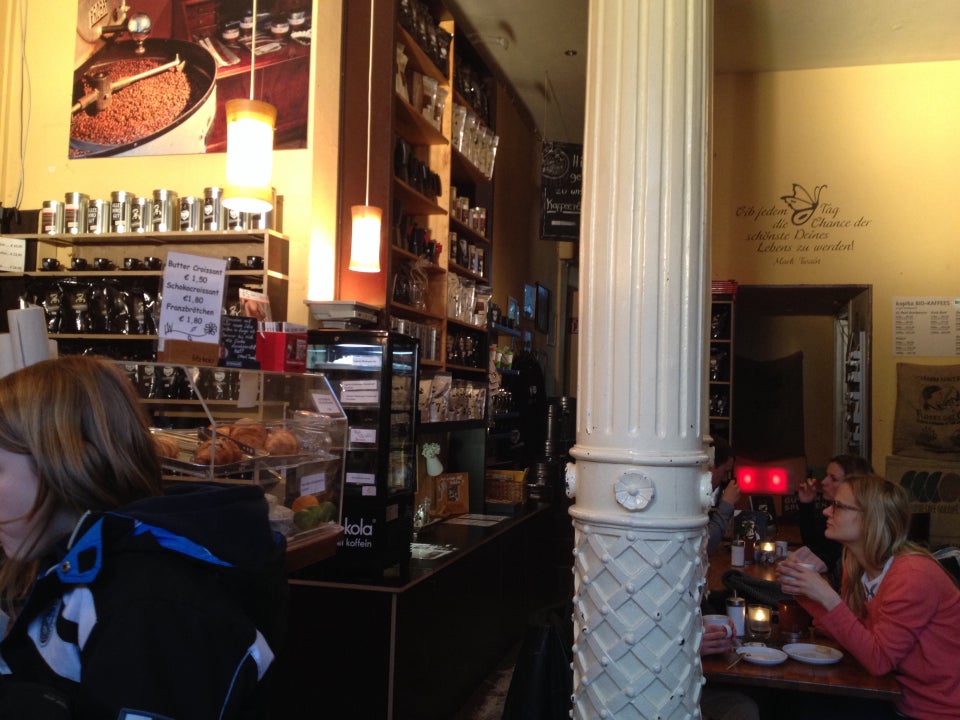This detailed photograph captures the cozy, well-lit ambiance of a small coffee shop. The central and left walls form a right angle, with the left wall painted yellow and the middle wall a rich brown. Both walls are adorned with shelves holding clear containers with labels, silver-topped jars, black coffee mugs, and an assortment of glassware. Notably, the left wall features a display case with an assortment of pastries, including a sign indicating "Butter Croissant $1.50". 

In the foreground, on the lower left, a young woman with brown hair, dressed in a blue, white, and black jacket, is partially visible. The room is defined by a tall, white central pillar with vertical grooves on the upper part and a crosshatched diamond pattern on the lower section, topped with a floral emblem.

On the right, a young lady in a red shirt is seated, drinking coffee with several plates in front of her on a small table. A second young woman is partially visible to the left, just her face seen. The background is somewhat shadowed but contrasted with the brighter areas near the yellow wall, which has some writing on it and leads to a back room through a doorway.

Multiple cylindrical lights with yellow casings hang from the ceiling, casting a warm glow over the scene. The setting is rich with coffee-related items, including cups, bottles, and various accessories for drinking and eating, creating an inviting atmosphere bustling with activity.